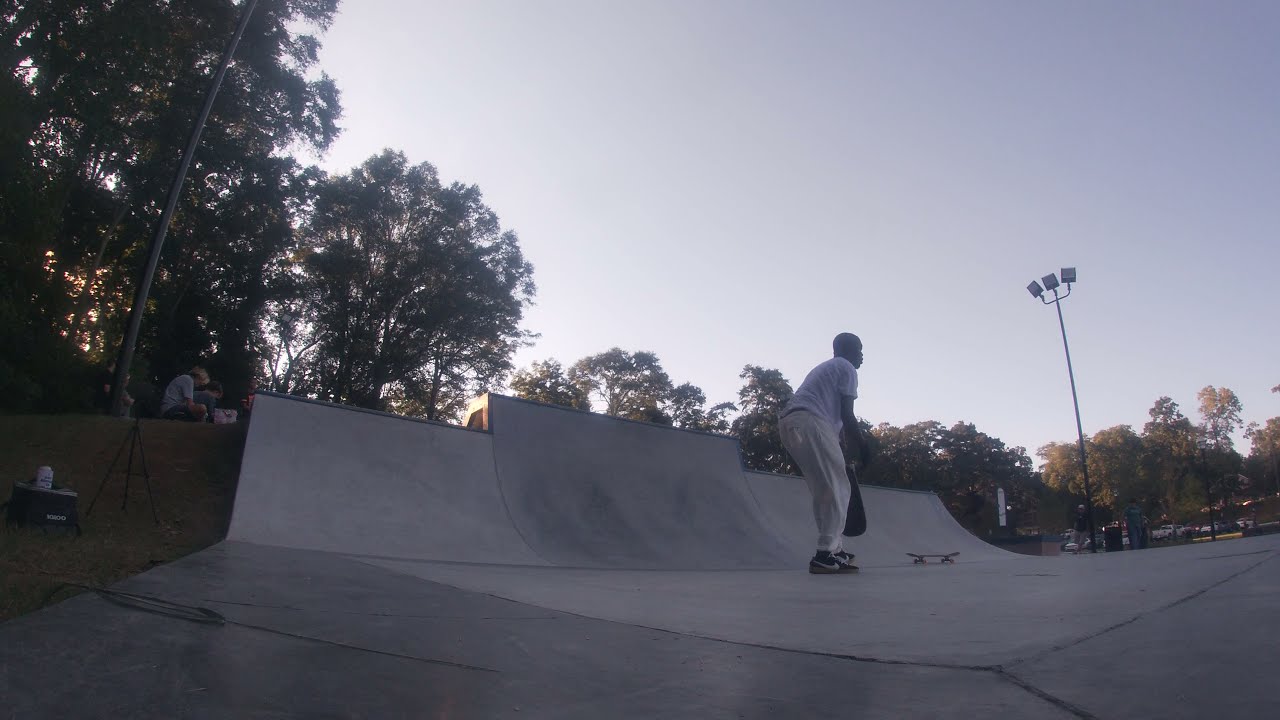In this detailed, full-color landscape photograph taken outdoors during sunset, a blue sky occupies the upper right corner, transitioning to a shaded foreground. The scene is set in a skatepark with a concrete surface and various ramps, half-pipes, and platforms. Centered in the image is a young man, facing away to the right, wearing a white short-sleeve shirt, white long pants, and dark Nike shoes. He appears bent over, holding a bag, and is standing on a skateboard, with another skateboard lying nearby. To his left, a couple of ramps are visible, leading off into the distance. The background is lined with trees, and a floodlight stands unlit in the right center of the frame. On the far left, next to the trees, a couple of individuals are seated on the grass near a tripod, possibly having a picnic. The overall atmosphere is tinged with the golden hues of the setting sun, casting a serene yet dynamic mood onto the skatepark.